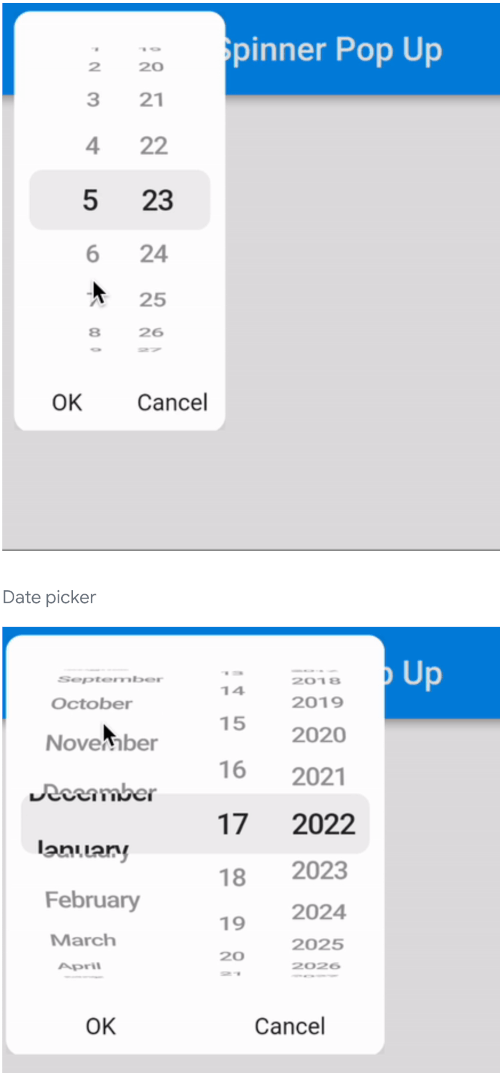A detailed screen capture showcases an interactive interface possibly from a mobile phone. At the top, there’s a section with a blue border labeled "Spinner Pop-up", transitioning to gray at the bottom. This section features a secondary white rectangle on the side which contains numerical selectors with numbers displayed on the left and right. The user has selected the numbers "5" and "23". Beneath this, there are two buttons labeled "OK" and "Cancel".

Separated by a white border, below lies another interface element labeled "Date Picker". The top of this section is also blue, with a partially visible label that reads "up". A prominent white square covers most of this area, likely listing selectable dates. The date selection tool displays a month on the left, a day in the center, and a year on the right. Currently, it seems to visually balance between December and January, with the selected date being "17" and the year "2022".

At the very bottom of the date picker, there are again options to confirm or cancel the selection, with "OK" to the left and "Cancel" to the right. The background behind this interface is gray, providing a neutral backdrop with no additional text or images visible below this point.